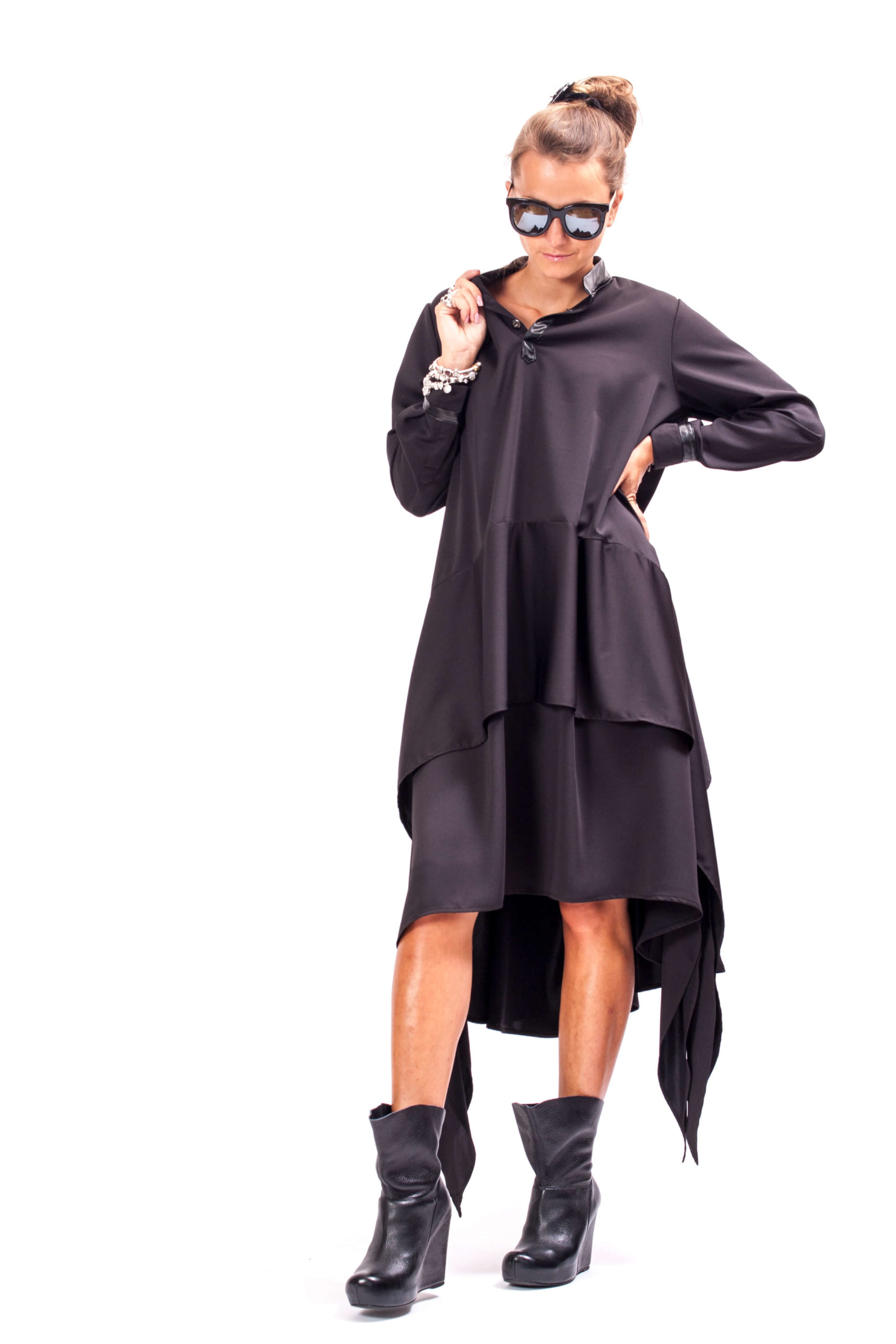In the image, a white woman stands confidently against a solid white background. She dons a loose-fitting, light brown long-sleeve dress that extends to her wrists and features a unique design—ending just below her knees in the front and dipping lower at the back with a tail-like section on the right side. Her light brown hair is pulled back into a bun, and she accessorizes with striking dark black sunglasses with silver reflections on the rims. Her right hand, adorned with white-colored bead bracelets, is raised above her shoulder, while her left hand rests on her hip. Both of her legs, visible from the knees down, catch subtle white reflections. She completes her outfit with black, heavy, high-top boots that are loose around her ankles and feature flat heavy platforms. Her composure radiates through her downturned face with pursed lips, adding an air of introspection to her poised stance.